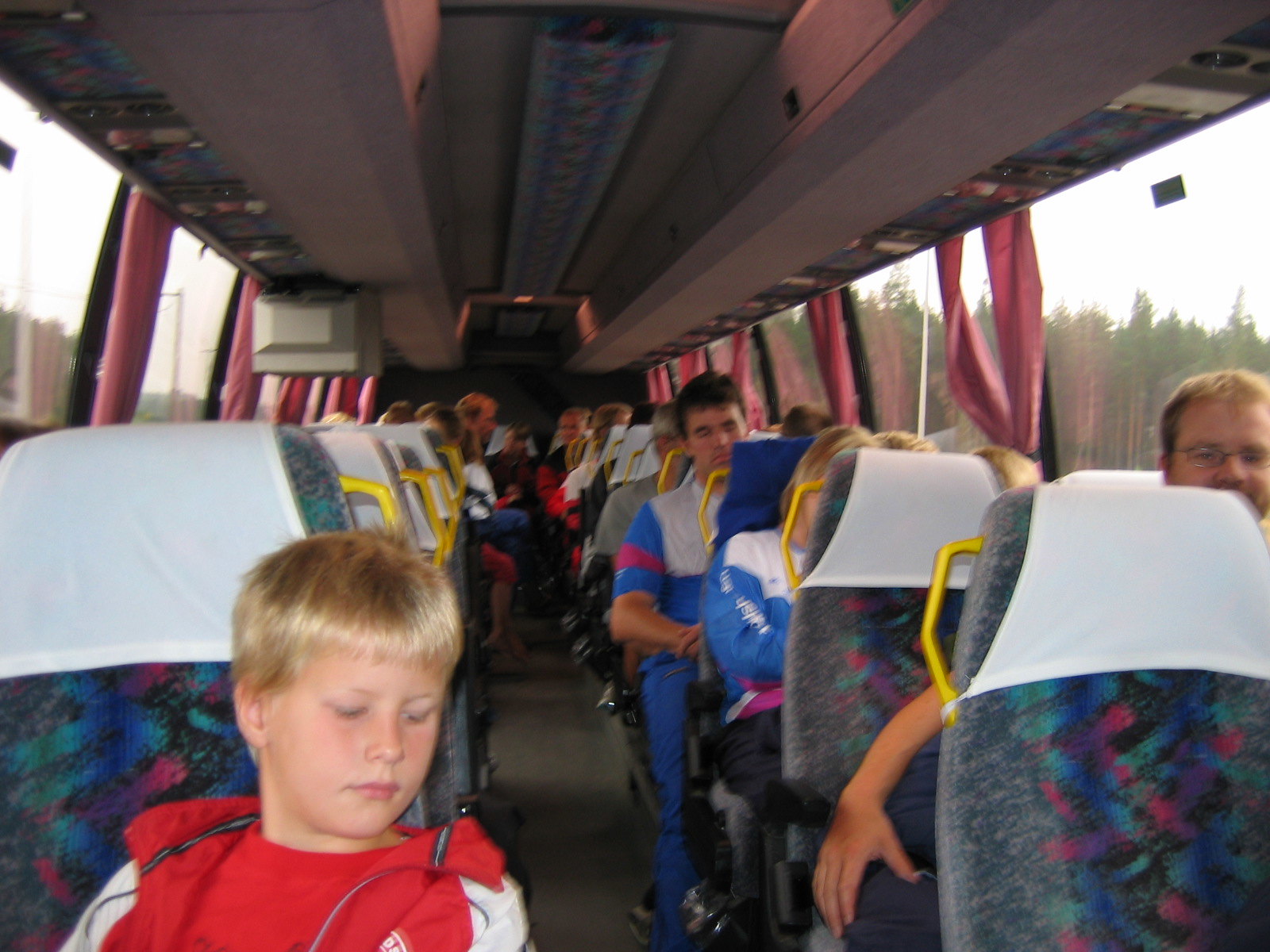The photo captures the interior of a bus, possibly a charter or tour bus, looking from the front towards the back. The seats are mostly filled, predominantly with adults, but there are a few children visible. The seats are black charcoal with a geometric pattern comprising blue, green, and red designs, along with some yellow flecks. Each seat is equipped with a white cloth covering the headrests and a bright yellow metal handle. 

In the front left seat sits a young blonde boy, approximately 10-12 years old, with a bowl cut hairstyle. He wears a red shirt and a red and white jacket, and his eyes are closed as if he is sleeping or looking down. Behind him, seating appears less occupied immediately, but gradually fills towards the back of the bus. On the right side of the front row, a white man with glasses is visible, and behind him, a blonde woman whose face is obscured by the seat. More individuals can be seen scattered throughout the bus.

The bus has large windows on both sides, partially framed by pink curtains drawn back to reveal a view of coniferous trees outside. A long light fixture runs along the ceiling, and there's a TV mounted overhead near the front. The vibrant and somewhat dated interior design, coupled with the style of clothing, suggests that the photo was taken around 10-15 years ago.